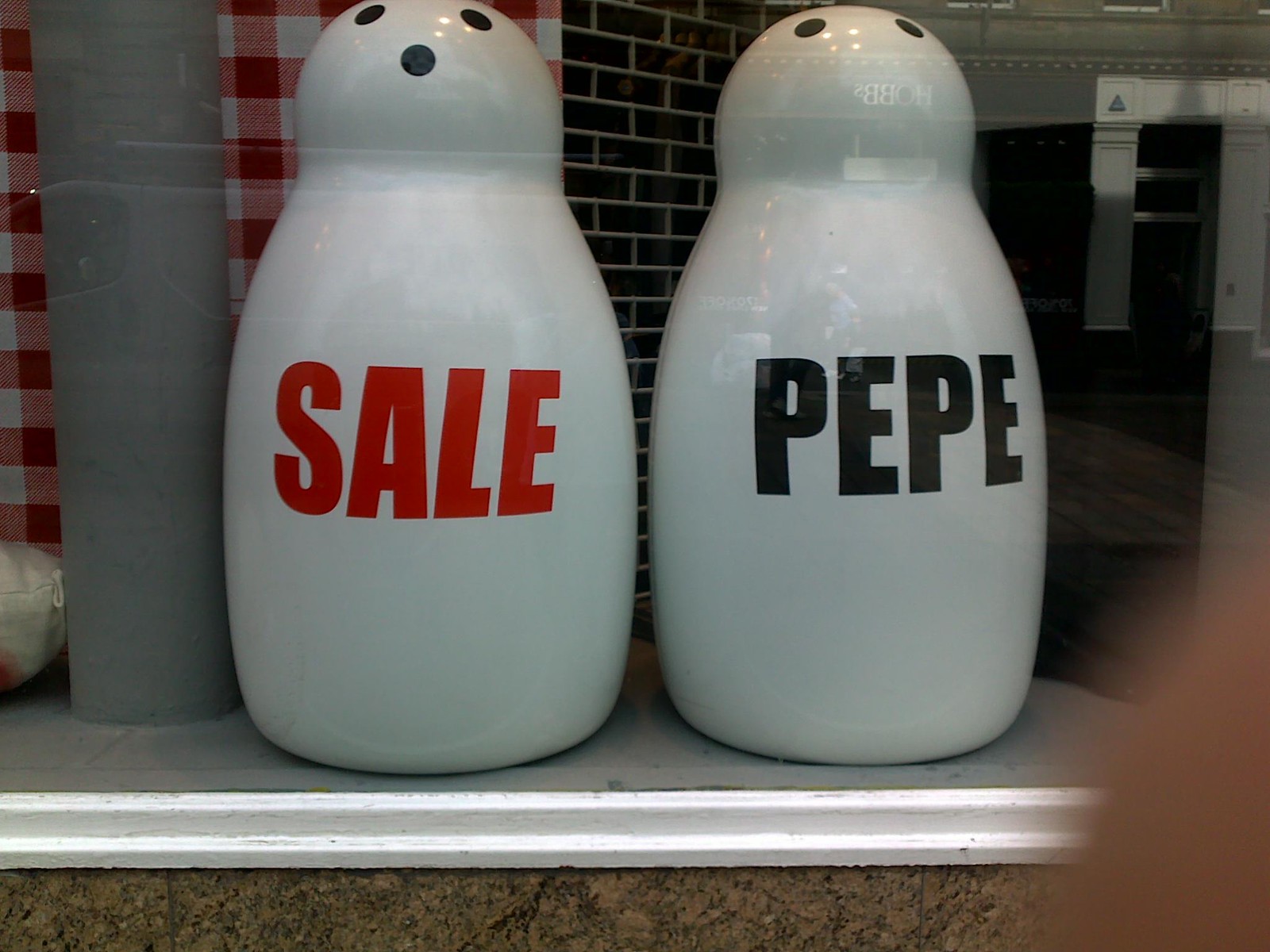The image depicts two large, white, shiny ceramic bottles, resembling oversized salt and pepper shakers, positioned on a white shelf. Both bottles have a rounded top and a long body, with a high-gloss finish. The bottle on the left, marked with the word "SALE" in red capital letters, features three black holes at the top. The bottle on the right, labeled "PEPE" in black capital letters, has two black holes at the top. The objects are likely decorative rather than functional, given their size and solid appearance. The scene is set behind glass, as evidenced by the reflections of light and images from the outside. Background elements include a black brick wall and a red and white checkered pattern, with additional details like a silver cylinder and potential finger blur at the bottom right corner of the image, suggesting the picture was taken indoors with some outside reflections visible.